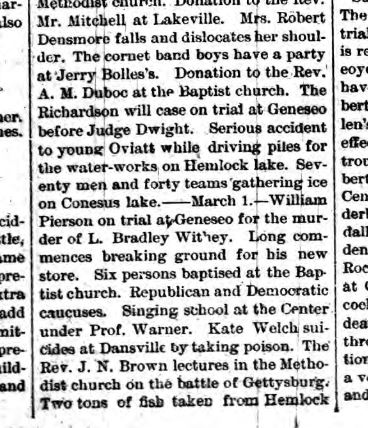The image captures a black-and-white section from a newspaper, featuring a clearly legible middle column while the left and right columns are cropped and illegible. The middle column, bordered by thin black lines, includes various local news snippets: "Mr. Mitchell at Lakeville. Mrs. Robert Densmore falls and dislocates her shoulder. The Cornet Band Boys have a party at Jerry Bolland's. Donation to Rev. A.M. Dubu at the Baptist Church. The Richardson case on trial at Geneseo before Judge Dwight. Serious accident to young Ove Lott while driving piles for the waterworks on Hemlock Lake. 70 men and 40 teams gather ice on Conesis Lake. William Pearson on trial at Geneseo for the murder of L. Bradley. Six persons baptized at the Baptist Church. Republican and Democratic caucuses. Singing school at the Center under Prof. Warner. Kate Welch suicides at Danville by taking poison. Rev. J.N. Brown lectures in the Methodist Church on the Battle of Gettysburg. Two tons of fish taken from Hemlock." The content details various events and incidents in a small town, providing a snapshot of everyday local happenings.